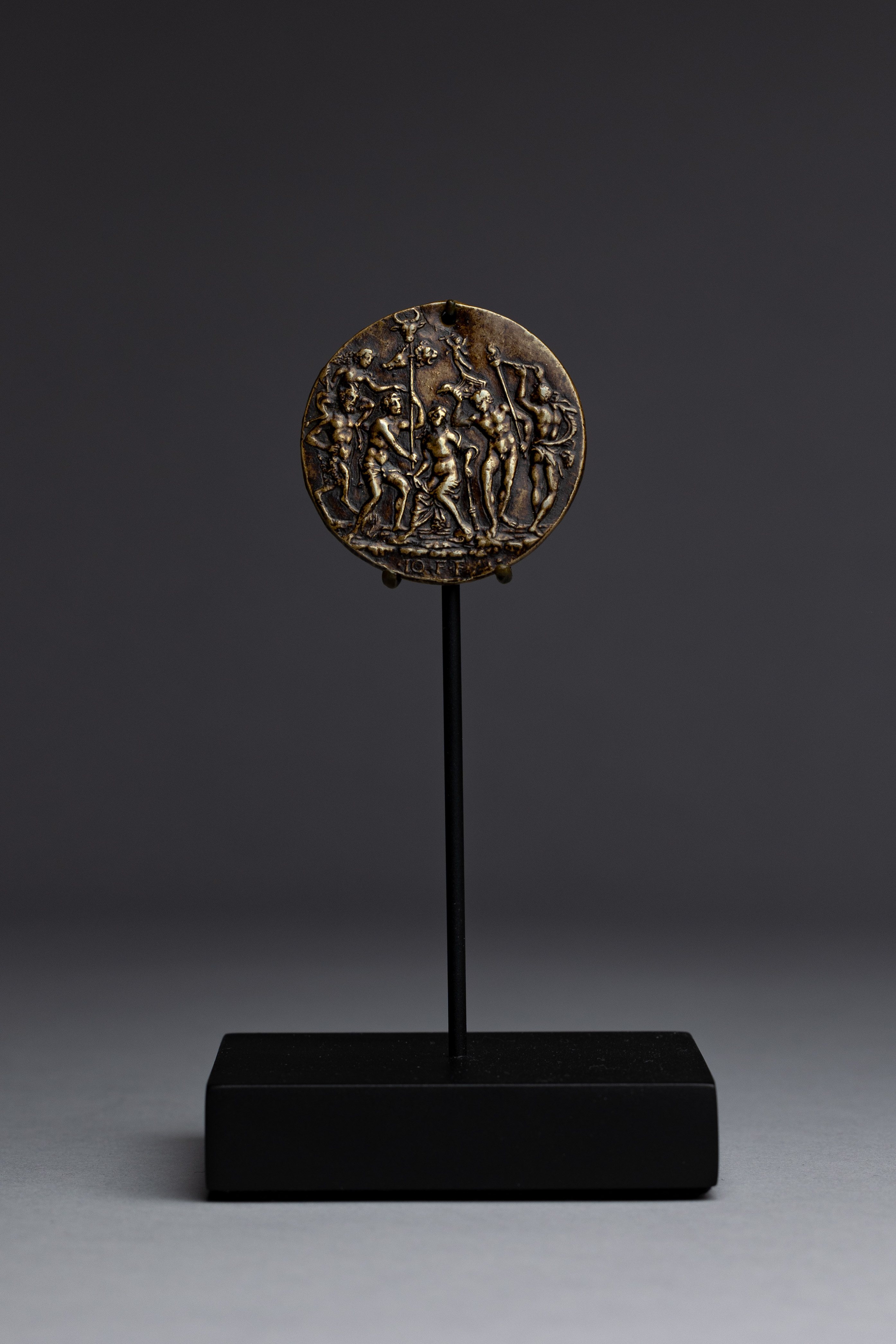The image depicts a small sculpture set against a neutral gray background. The sculpture features a rectangular black base that appears heavy and is likely made of metal, stone, or marble. From the center of this base, a slender black metal rod rises vertically. At the top of the rod is a bronze-colored circular medallion adorned with intricate golden engravings. These engravings depict several almost naked human figures, both men and women, who are closely positioned and holding sticks or rods. Some figures also appear to have robes draped over their shoulders. The medallion has an ancient, possibly historical appearance, further emphasized by its detailed artwork. The entire composition is isolated with no other objects, allowing full focus on the sculpture itself.